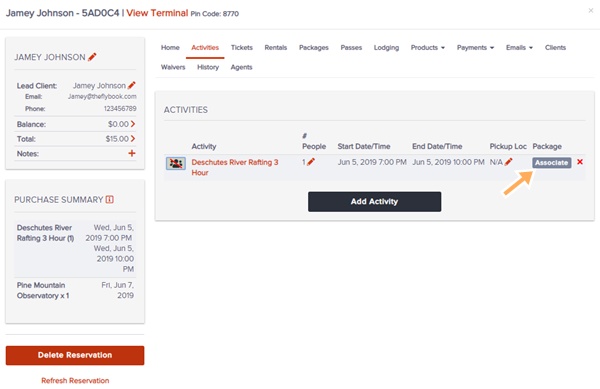**Screenshot of a Web Page Interface**

The screenshot displays a webpage layout featuring various UI elements designed for user interaction. On the left side, there are two distinct, square-shaped grayed-out sections. The upper square section displays the name "Jamie Johnson," while the lower square section is labeled "Purchase Summary."

To the right of these sections, there is a wide, horizontal rectangle also shaded in gray, with a subtle drop shadow applied to all these shapes, adding a slight 3D effect. Above this horizontal rectangle, lies a navigation menu formatted as a horizontal strip of hyperlinked items with the following labels, from left to right: "Home," "Activities" (highlighted in red with an underline), "Tickets," "Rentals," "Packages," "Passes," "Lodging," "Products" (accompanied by a downward-pointing arrow), "Payments" (with a downward-pointing arrow), "Emails" (with a downward-pointing arrow), "Clients," "Waivers," "History," and "Agents." 

The terms "Products," "Payments," and "Emails" each have accompanying downward-pointing arrows indicating dropdown menus. Beneath the main menu bar, the labels "Waivers," "History," and "Agents" are also present in a secondary menu section starting just below "Home."

Further down, beneath the "Purchase Summary" section, there is a red, horizontally-aligned box with white text that reads "Delete Reservation." Below this button, another text labeled "Refresh Reservation" appears in red.

The overall interface suggests a detailed user account or reservation management system, providing multiple navigational and action-oriented options for the user.